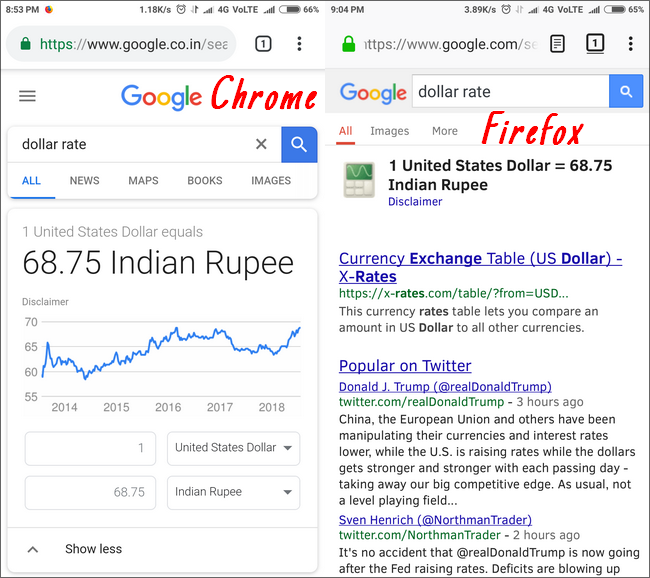The image is a comparative screenshot of two mobile phones displaying currency conversion results on a search engine, against a white background. The image is divided vertically by a thin gray line. 

**Left Side:**
- At the very top is a search bar with "google.com" on its right.
- Below it, there is an icon featuring three horizontal black lines to the left and a square with the digit '1' and three vertically arranged dots to the right.
- The center displays the Google logo, beneath which is "Chrome" in red text.
- Below the logo, a search bar contains the query "dollar rate" with a blue square and white magnifying glass icon on its right.
- Under the search bar, there are navigation options: "All" in blue, followed by "News," "Maps," "Books," and "Images" in black text.
- Further down, the conversion result states: "1 United States Dollar equals 68.75 Indian Rupee" in large lettering. Below this is the word "Disclaimer."
- A graph on the left side indicates fluctuating currency rates, with vertical markers at 70, 65, 60, and 55, and horizontal markers showing the years 2014 to 2018. The blue line on the graph shows the trend across these years.
- At the bottom of the graph are four rectangles; the top left says “1,” the bottom left says “68.75,” the top right indicates "United States Dollar," and the bottom right shows "Indian Rupee." The bottom left corner has the text "Show less" in black.

**Right Side:**
- The setup is mostly similar to the left side but with notable differences.
- Here, the Google logo is to the left, and the browser indicated in red text is "Firefox."
- The search query "dollar rate" remains the same, with the blue square icon on the right.
- Navigation options are displayed slightly differently with "All" in red and "Images" and "More" in black text.
- The conversion result is bolded: "1 United States Dollar equals 68.75 Indian Rupee," followed by "Disclaimer."
- Additionally, two blue clickable links are presented, the first accompanied by a paragraph of information and the second by two paragraphs.

This detailed comparative display elucidates the appearance and results of a basic currency query on two different browsers, highlighting both functional and aesthetic elements.